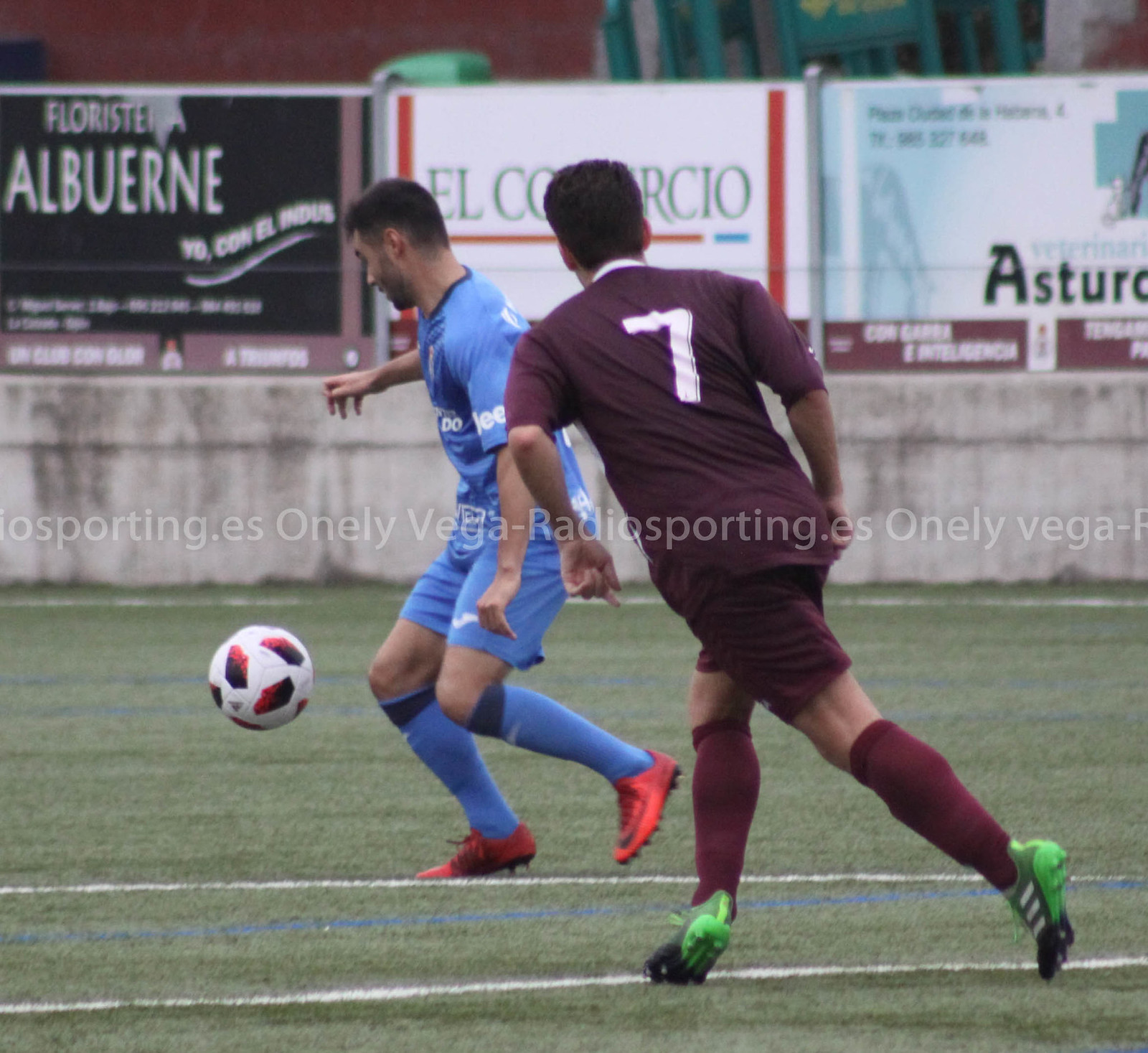This vibrant outdoor photograph captures an intense soccer match during the day, set on a green field adorned with white and blue markings. The dynamic scene focuses on two men, who appear to be of Hispanic descent, competing for control of a white soccer ball decorated with red and black graphics. The player in the foreground is captured mid-kick, wearing a light blue jersey, shorts, and socks, complemented by red cleats. His dark hair adds to his focused demeanor. Hot on his trail is another player in a striking maroon uniform, complete with maroon shorts, socks, and green and gray adidas cleats, emblazoned with the number 7 in white on his back. The backdrop features a weathered concrete wall adorned with several billboards displaying text in a foreign language. The most discernible ads include one with white lettering "A-S-T-U-R-C," another partially obscured ad starting with "E-L" and ending in "C-O-R-I-C-I-O," and a black ad with "A-L-B-U-E-R-N-E" in bold white letters, conveying the spirited amateur ambiance of this local match.